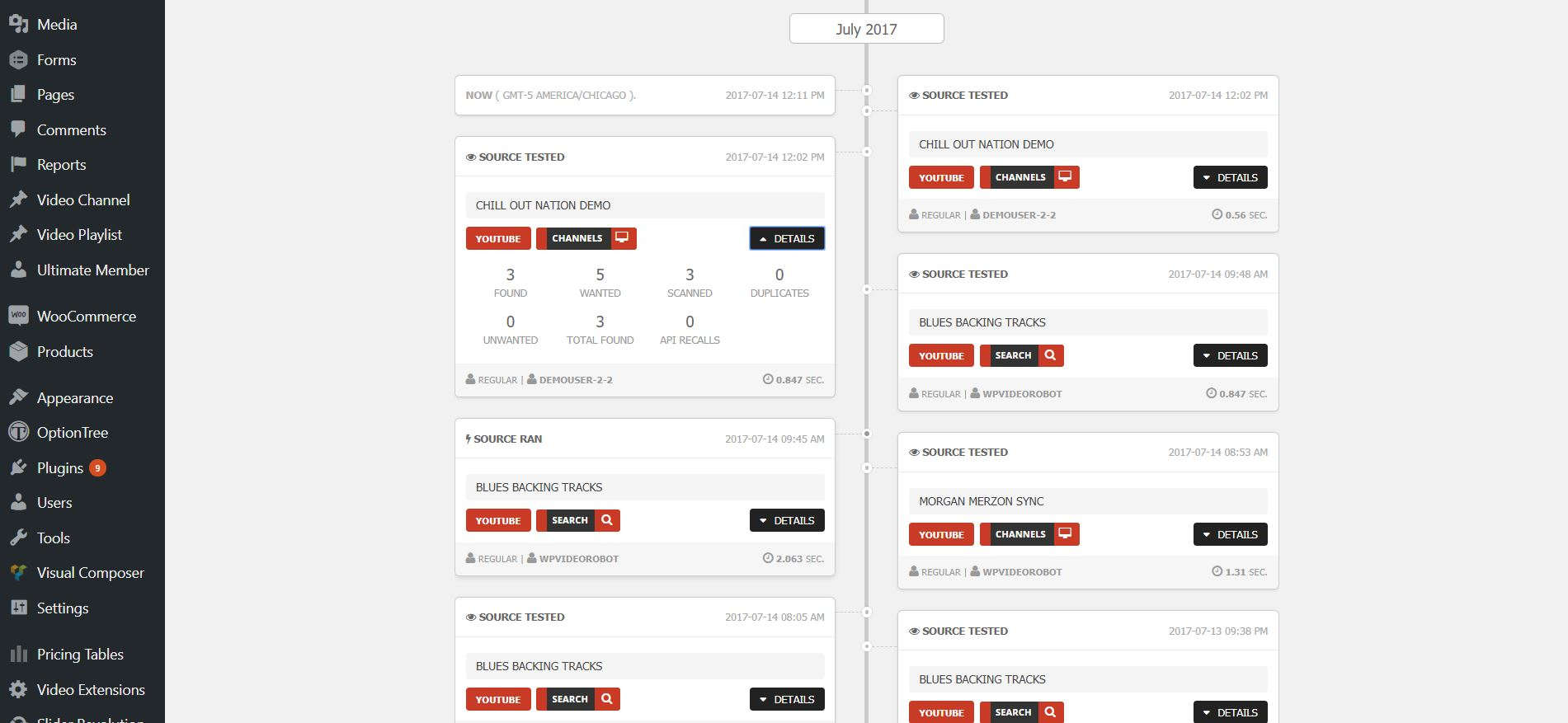The image depicts a screenshot of a highly detailed interface, though it is too small to read clearly. On the left side, a menu with large grey options is displayed, each adorned with small icons. These options include "Media," "Forms," "Pages," "Comments," "Reports," "Video Channel," "Video Playlist," "Ultimate Member," "WooCommerce," "Products," "Appearance," "Entries," "Plugins," "Users," "Tools," "Visual Composer," "Settings," "Pricing Tables," and "Video Extensions." To the right of this menu, there is a date listed as July 17th, followed by a vertical bar.

There are several tabs resembling rectangles arranged on either side of the screen, providing information in a structured manner. However, the small size of the images renders the text unreadable. Some red fields with icons, potentially screens and search bars, are scattered throughout the interface—approximately 2 or 3 on the left and another 4 on the right, originating from various sections. A vertical timeline is present, although its purpose remains unclear. Each rectangle on the right includes black detail buttons with white text, but the overall clarity of the screenshot is severely compromised by the tiny image size, making it difficult to discern any specific details.